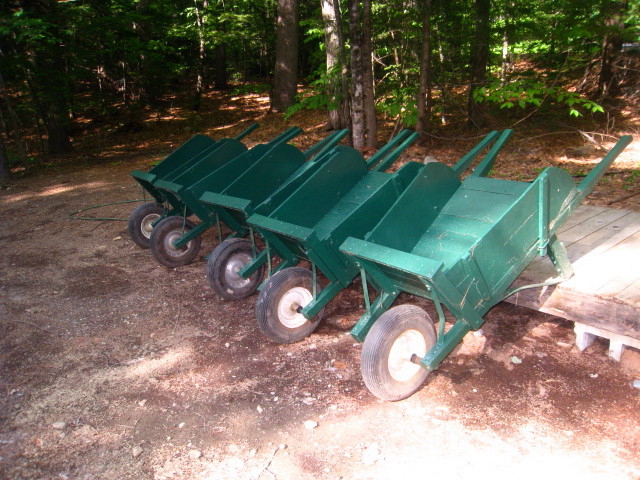The photo captures five identical green wheelbarrows, each with a single black wheel featuring a silver or white hubcap. Lined up in a neat row from right to left, the wheelbarrows have rectangular, wooden bodies with open ends closest to their green-painted handles and rails. Propped up on a long, weathered wooden boardwalk supported by cinderblocks, the scene includes a dirt ground scattered with rocks and small twigs. In the midst of this outdoor setting, a green hose is visible to the left of the wheelbarrows. The background reveals a mix of deciduous trees, with sunlight filtering through the foliage, hinting at a forested area or park with a trail leading off into the distance.